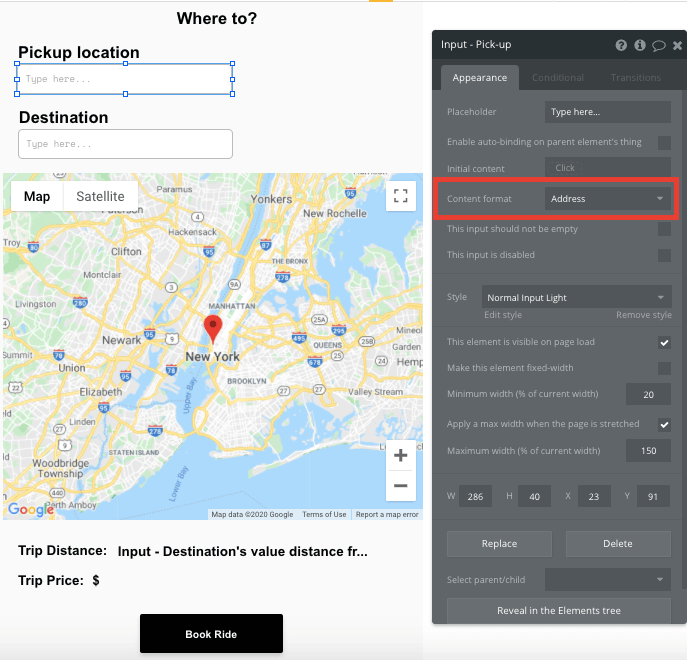This image, captured from a website interface, features a structured layout designed to facilitate booking a ride. At the top, there's a header containing a partially obscured query indicated by "where to question mark." Below this, on the left side, there are labeled input fields: one for entering the "Pick Up Location" and another for the "Destination." 

Directly beneath these input boxes, a map is prominently displayed, centered on New York City and marked with a red pin. Beneath the map, there are fields labeled "Trip Distance," which displays the calculated travel distance, and "Trip Price," which shows the cost in a monetary format, both followed by ellipses indicating incomplete information.

At the bottom left, a black button with white text reads "Book Ride," suggesting an actionable step for users. Adjacent to the map, on the right side of the layout, a gray section houses a format validator for input addresses. This section is highlighted by a red outline and contains messages including "This input should not be empty" and "This input is disabled." Below these messages, there's a style option indicated as "Style: Normal Input Light," followed by a list of configurable settings.